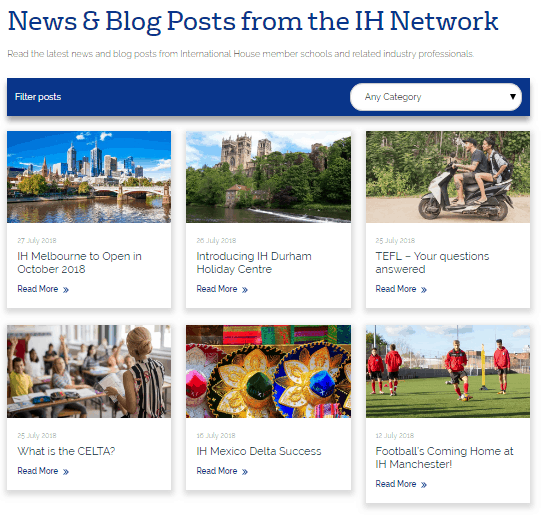This is a screenshot of a website with a clean, white background. At the top of the page, there is a bold headline in navy blue font that reads "News and Blog Posts from the Hi-H Network." Below this, a smaller text provides further context: "Read the latest news and blog posts from international house member schools and related industry professionals."

Directly beneath this text is a navy blue navigation bar. Towards the right side of this bar, there is a small white oval-shaped drop-down menu with the text "Any Category" in black font. On the left side of the bar, it displays "Filter Posts."

Further down the page, there are two rows of entries, with three entries per row, making a total of six entries. Each entry consists of a square divided into two halves: the upper half features a small picture, and the lower half is a white bar containing text.

Starting from the upper left, the first entry displays a photo of a city taken from across the water, featuring a bridge and two prominently visible skyscrapers. Beneath the photo, in grey font, the date "27 July 2018" is displayed. Below the date, in black font, it reads "IH Melbourne to open in October 2018."